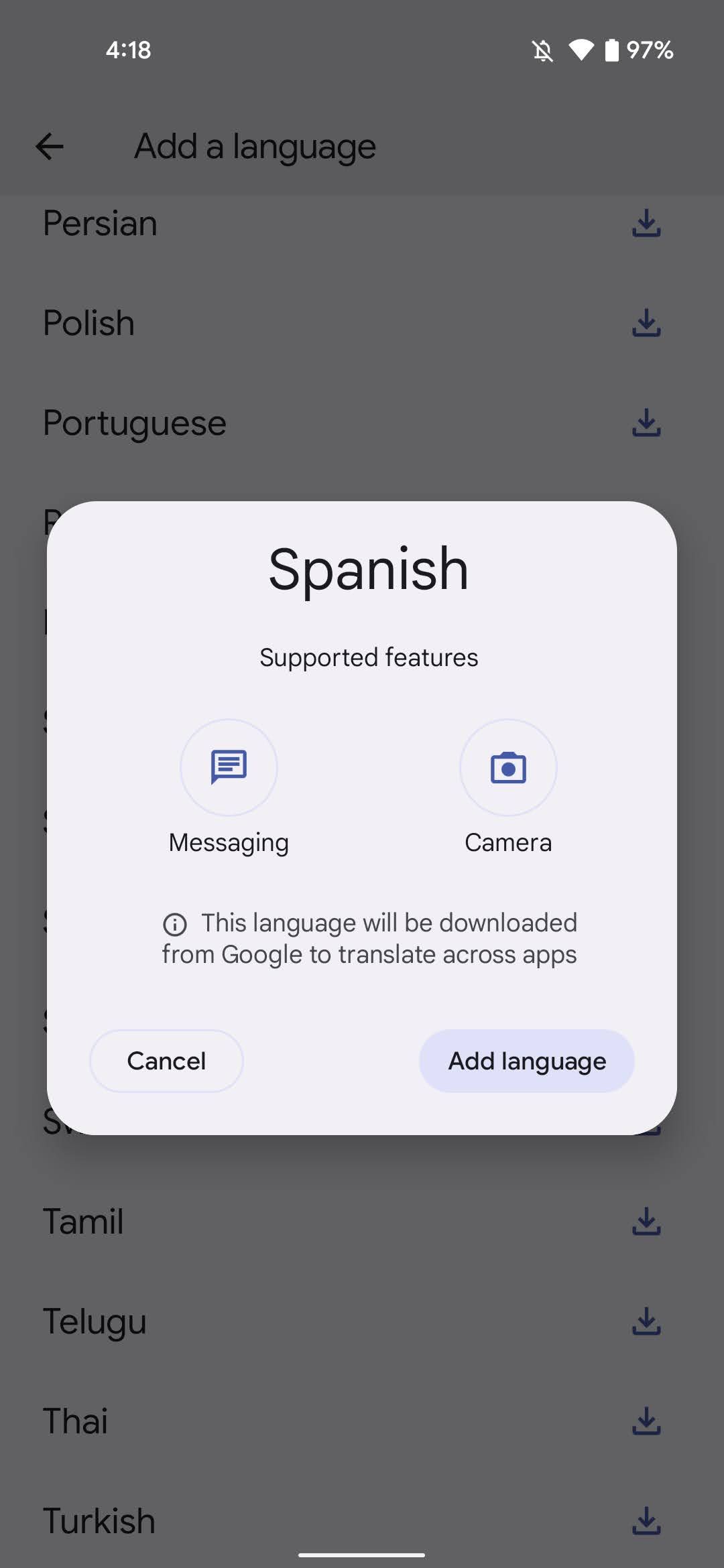This image features a phone application interface focused on language selection. The app's layout prominently displays a section mostly grayed-out, except for a highlighted white square at the top that currently shows the language “Spanish.” Available language options presented include Persian, Polish, and Portuguese, while Tamil, Telugu, Thai, and Turkish are shown as unavailable and grayed-out. Beneath the language options, detailed features supported by the selected language are listed, such as messaging and camera functionalities. Additionally, a note indicates that "This language will be downloaded from Google to translate across apps." At the bottom of the interface, there are two actionable buttons: “Cancel” and “Add Language.”